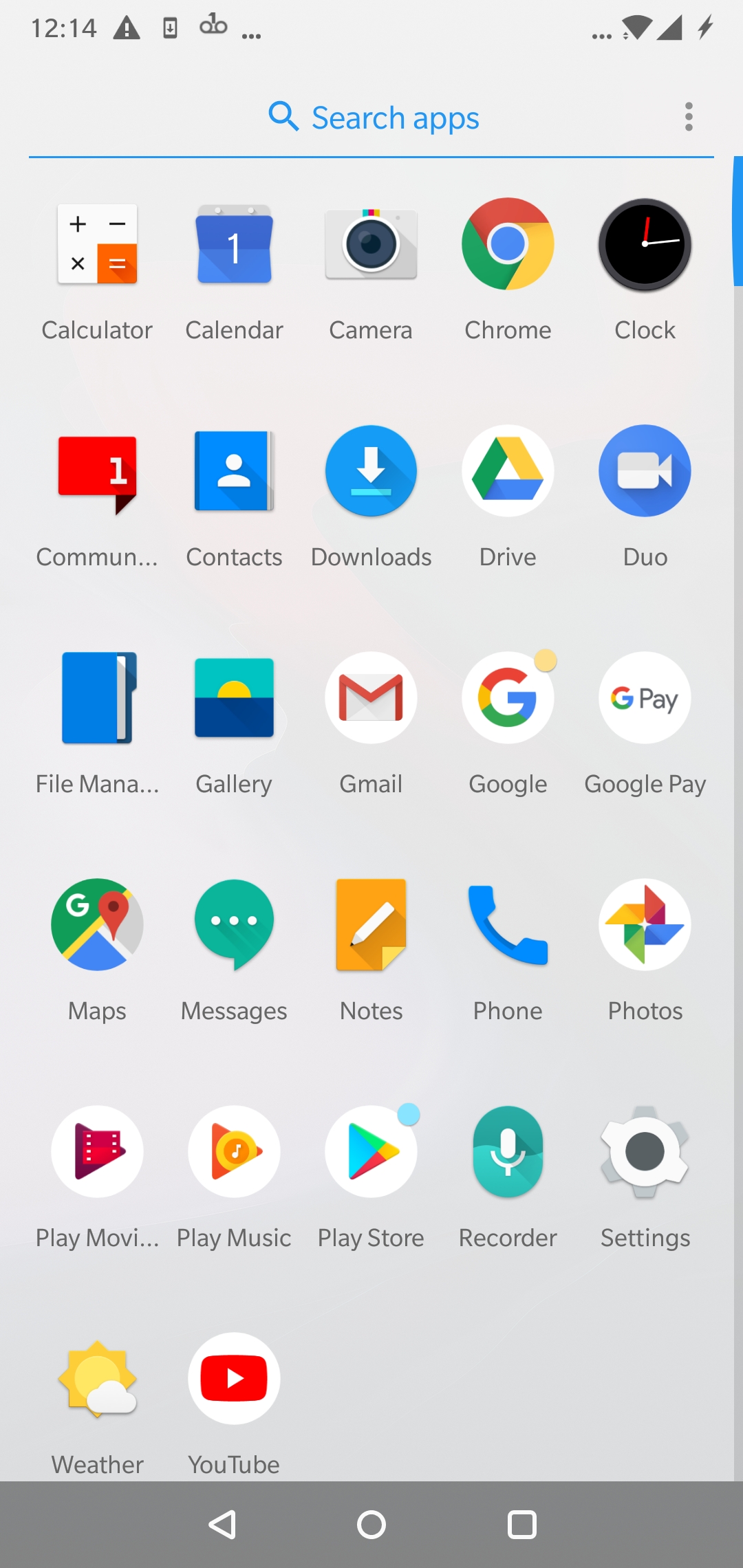The image displays the app drawer of an Android phone, featuring a collection of default applications that typically come pre-installed. The background is a light gray hue, providing a neutral setting that highlights the app icons. Most of the icons are circular, though some deviate into square or rectangular shapes. Among the visible apps are essential tools like Calculator, Calendar, Camera, Clock, Contacts, Downloads, and essential Google apps such as Chrome, Drive, Duo, Gmail, Maps, Messages, Play Store, and YouTube. Additionally, utility apps like File Manager, Gallery, Notes, Phone, Recorder, Settings, and Weather are also present. Several icons have small badges or dots, possibly indicating unread notifications or updates. The notification bar at the top displays a lightning bolt, which might signify that the device is currently charging. There are also small icons near the top, depicting either a bicycle or glasses, though their specific meaning is unclear.